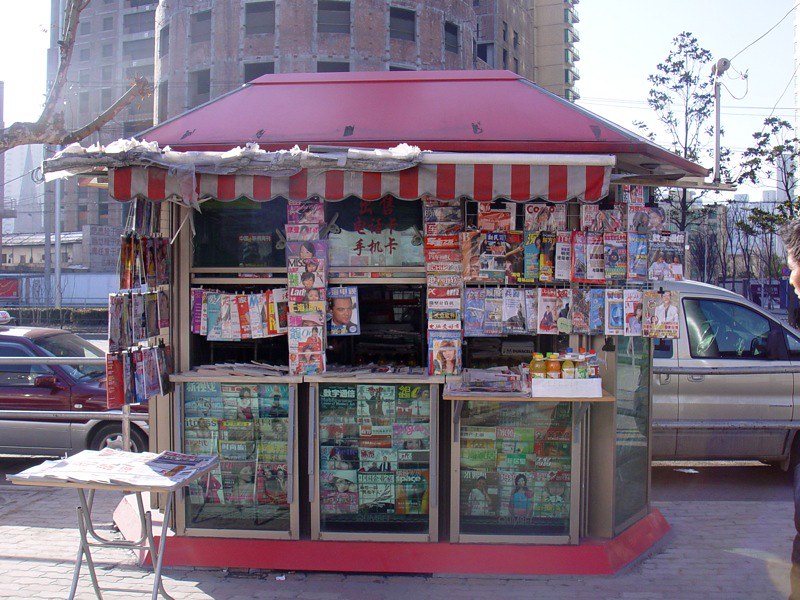This photograph captures a bustling newsstand situated on the side of a street, featuring a distinctive red base and a slanted red roof complemented by a red and white striped awning. The newsstand's exterior is lined with glass windows displaying an array of magazines, many of which hang in front of the windows, while others are behind the glass or placed on a fold-out tray table outside. The majority of the print on the magazines appears to be in Japanese, though there are also some English titles. Inside the kiosk, which is typically found in a large city, there are also juices and cigarettes for sale. In the background, there is a steel gray railing, along with a building made of reddish-brown brick. Additionally, there are other buildings featuring balconies and windows, and some trees flanking both sides of the scene. On the street, to the left, there is a two-tone car with a red top and silver bottom, and to the right, a tan-colored car, adding to the urban atmosphere.